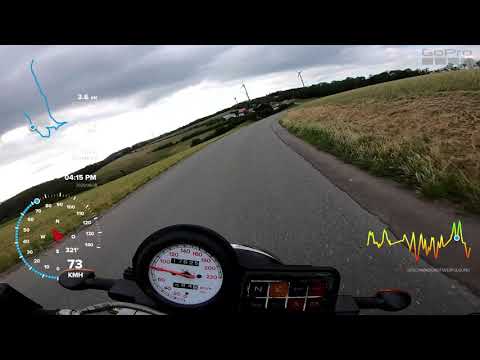The image depicts a motorcyclist taking a photo while riding on a winding road, captured through a GoPro camera. The sky is dominated by gray clouds, creating a moody atmosphere. The motorcyclist is traveling on a road flanked by green fields on both sides, with windmills visible in the distance. The foreground shows the motorcycle's handlebars and a speedometer displaying a speed of around 72 to 74 miles per hour. The GoPro logo is prominently displayed in the top right corner, and a colorful graph—yellow, red, and green—along with a map displaying a blue line, is visible on the screen, suggesting a combination of real-time data and possibly an augmented reality display. Scattered houses, telephone poles, and power lines can be seen on the horizon, indicating a semi-rural setting. The overall scene blends the thrill of motorcycle riding with the advanced technology of the GoPro, capturing both the journey and the surrounding landscape in detail.